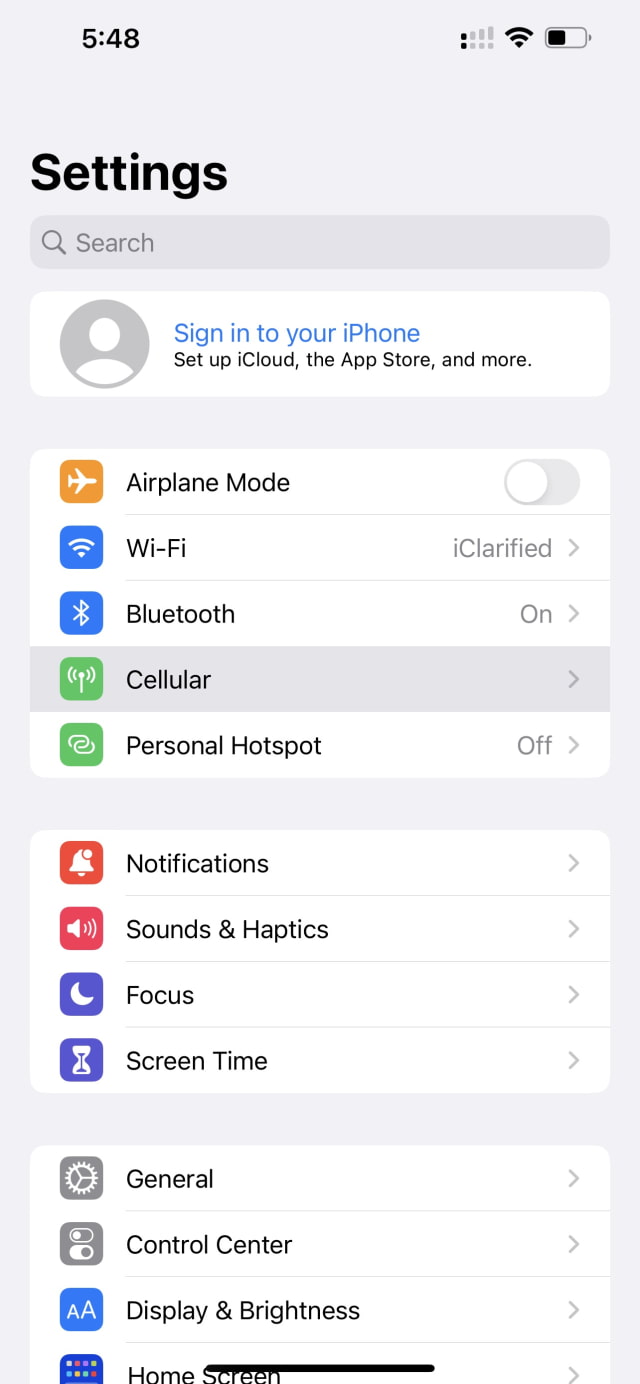This is a detailed screenshot of the settings page on a smartphone. The background of the page is predominantly grey, providing a neutral theme for the interface. At the top of the screen, prominently aligned to the left, is the title "Settings" displayed in large, bold text. Beneath this heading, there's a darker grey search bar allowing users to quickly search through the settings.

Immediately below the search bar, there's a white bar with the text "Sign in to your iPhone" featured in blue, next to the default profile picture avatar positioned on the left. This bar serves as a prompt for users to sign into their device.

Following this are three groups of settings, each organized within distinct white sections for better readability and interaction. Each section includes an icon on the left, the corresponding title next to it, and either a toggle switch or a forward arrow on the right to indicate further navigation or toggling.

The first group includes:
- **Airplane Mode** with a toggle switch,
- **Wi-Fi** with a forward arrow,
- **Bluetooth** with a forward arrow,
- **Cellular** with a forward arrow,
- **Personal Hotspot** with a forward arrow.

The second group consists of:
- **Notifications** with a forward arrow,
- **Sounds & Haptics** with a forward arrow,
- **Focus** with a forward arrow,
- **Screen Time** with a forward arrow.

This structured layout is designed to provide easy and quick access to various settings and configurations on the device.